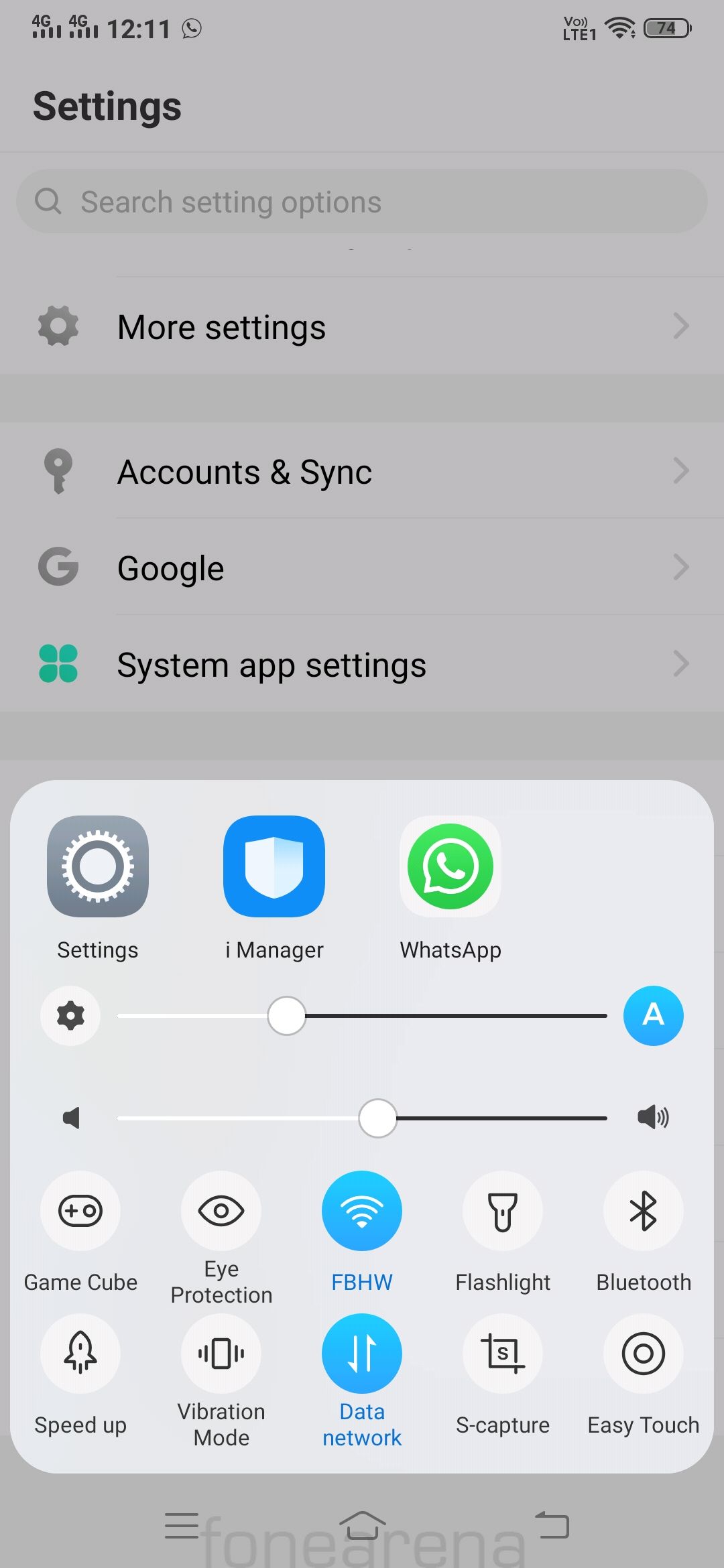The image showcases the settings page of a smartphone app, notably displaying various configurations and toggles. Towards the top left, the grey and white "Settings" option is prominently visible. Centrally located is the "iManager" icon, easily identifiable by its blue and white color scheme. Adjacent to this, the green and white "WhatsApp" icon stands out. Further down, a blue volume slider is shown, truncated halfway on the right side. Below this, a notification slider is depicted at half intensity.

Beneath the sliders, there is a series of toggle switches. From left to right, they start with "Gamecube," followed by "Eye Protection." The "FBHW" toggle, indicating Wi-Fi, is active, highlighted in blue. Next to this is the flashlight toggle, followed by Bluetooth. Continuing along the bottom row, there is the "Speed App," another toggle for vibration mode, and the "Data Network" toggle, also active and marked in blue. Concluding the row are switches for "S-Capture" and "Easy Touch," the latter positioned at the bottom right of the image.

In the image's background, a watermark at the bottom reads "Phone Arena." The upper portion of the background exhibits a search bar labeled "Search setting option." Below the search bar, various settings categories are listed, including "More Settings," "Account and Sync," "Google," "System," and "App Setting."